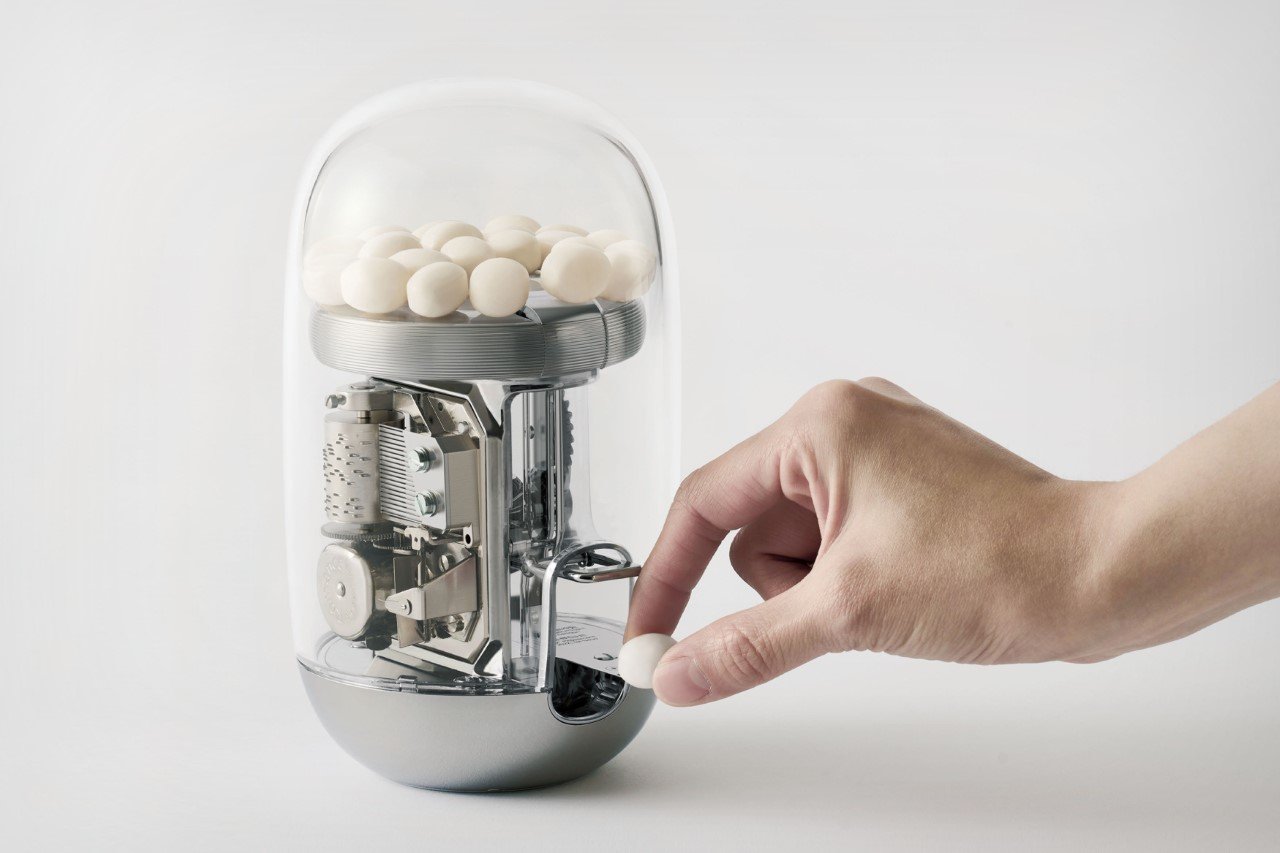In this detailed image, a uniquely designed candy dispenser, prominently shaped like a peel or pod, occupies the center stage against a gray-white background. The core structure of the dispenser consists of intricate mechanical wheels and pieces that intricately drop a white circular candy into the awaiting hand. Constructed with a clear plexiglass cover, the internal components and candies are visibly showcased, lending a sleek and transparent aesthetic. The device features a sophisticated metallic silver base, harmonious with the other silver elements that seem to hold the candy reservoir at the top. Multiple white candies rest on this metal plate, suggesting a plentiful reserve ready for dispensing. The image captures a hand at the moment of retrieving one dispensed candy, highlighting the machine's functionality and mechanical beauty. The subtle elements—such as the turn system, mechanical cord, and dull silvery finish—add to the intricate craftsmanship of the candy dispenser, firmly setting this photo as an indoor demonstration of its operational charm.